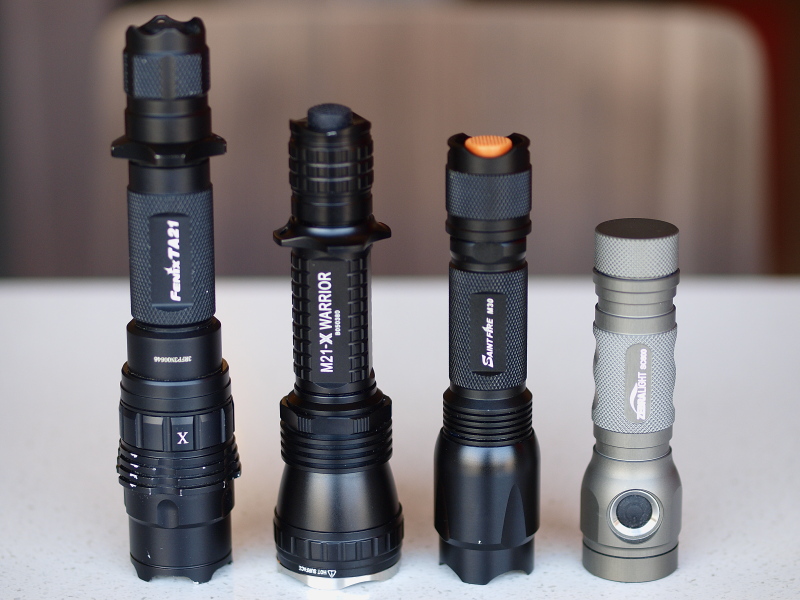The image captures a close-up of four flashlights arranged upright on a white table against a grayish background. The flashlights are organized from tallest to shortest, creating a descending order from left to right. The leftmost flashlight is black and features a label with unclear text, possibly "fend phoenix" or "ta ta to." It appears more robust and heavy-duty. The next black flashlight, slightly shorter, is identified as the "M21-X Warrior," denoting an advanced model. The third flashlight, also black but smaller, has an orange button on top and some indistinct white writing along its side. The final flashlight on the right is the smallest and is silver in color with a black button at the base near the light. It has a lighter gray strip in the middle and some white text. All the flashlights have their lens ends resting on the table, highlighting their vertical alignment.